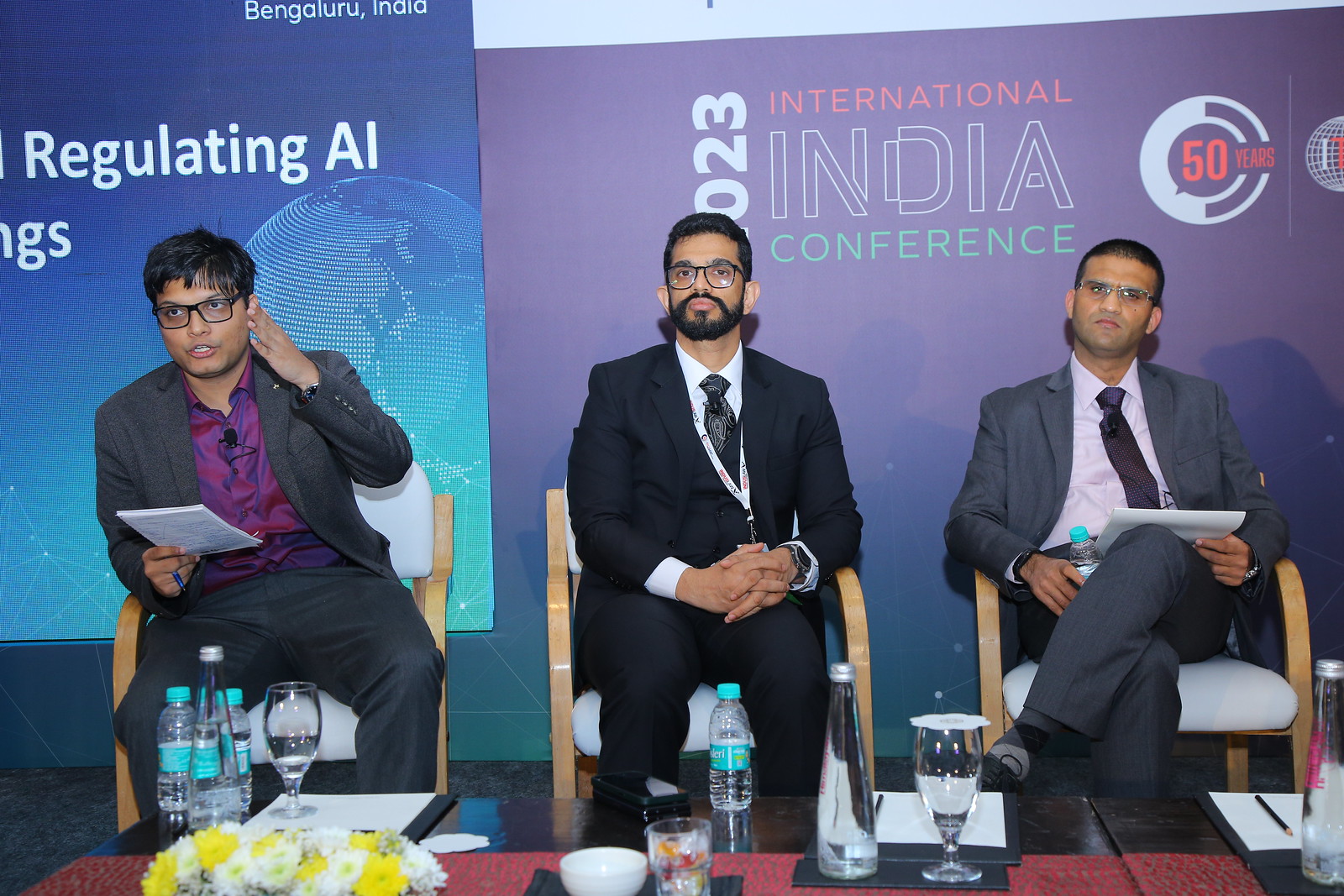The photograph captures a scene from the International Indian Conference 2023, a significant event themed around "Regulating AI," as indicated by the text on the backdrop. The setting is vibrant, dominated by a spectrum of colors including purples, blues, greens, dark blues, reds, whites, blacks, yellows, and lime greens.

The image features three Indian men, all seated in light wooden chairs with white cushions, positioned in the middle of the setting. They are dressed formally in suits: the gentleman on the left wears a gray suit with a bright purple shirt and no tie, and has a microphone affixed to his shirt. He is holding papers in one hand and has the other hand to his ear. The man in the center sports a black suit with a white shirt and a black tie, and has a mustache and beard. The gentleman on the right is attired in a gray suit with a white shirt and a dark-colored tie.

In the foreground, a table in front of the men is adorned with yellow and white flowers, water bottles, and glasses, adding to the conference ambiance. Behind the seated men are cardboard cutouts that contribute to the background décor. The overall presentation, including the floral arrangement, water glasses, and cardboard cutouts, enhances the formal and professional atmosphere of the event celebrating 50 years.